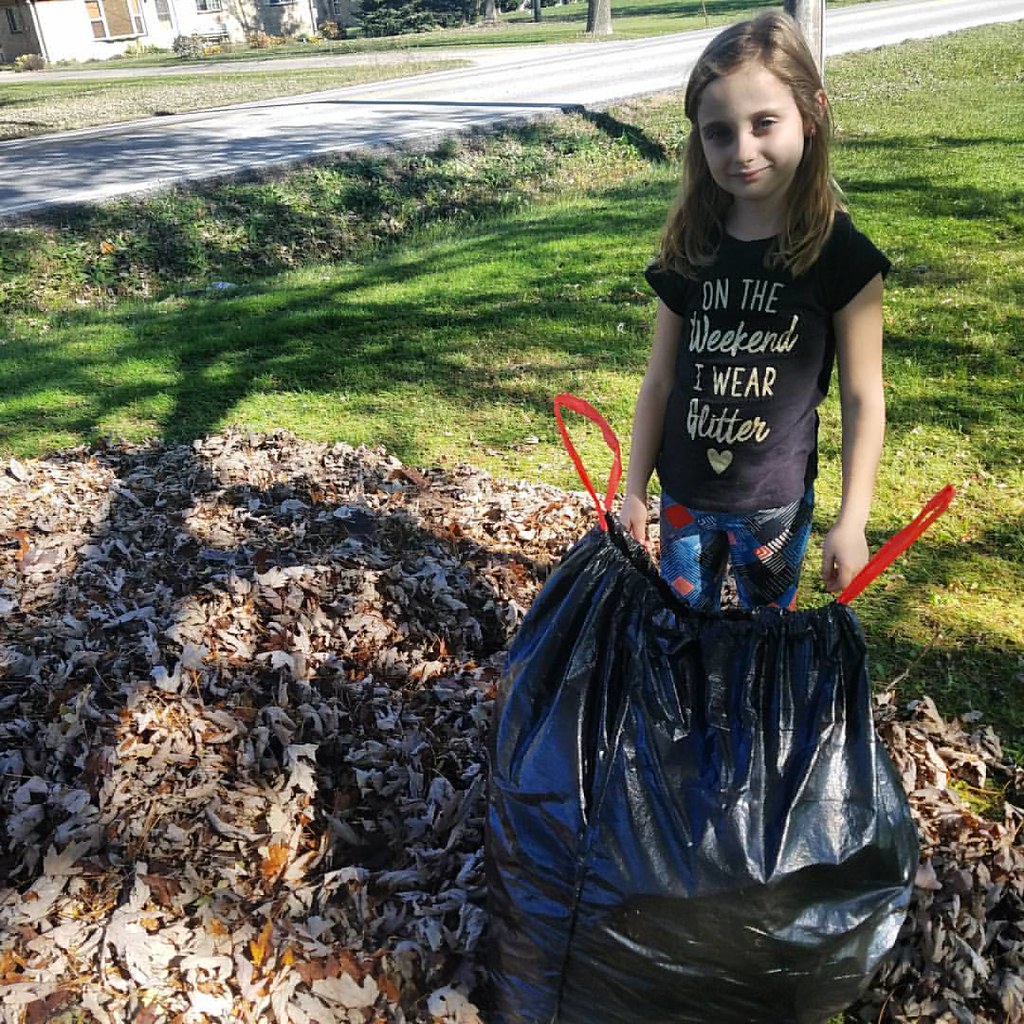The image captures a young girl standing amidst a large pile of brown fall leaves. She is smiling, though her smile has a hint of bitterness. Her head is tilted slightly to the left, and her brown hair, parted on the right, cascades down to her collarbone on the left side of her face. She is wearing a black t-shirt with the text "on the weekend I wear glitter" and a gold heart underneath. Her tight blue pants are adorned with different colored patches—red on the left side, and black with lines emanating from them on the right. The girl stands behind a big plastic trash bag with red strings, partway filled with leaves, implying she has been gathering them. Behind her stretches a green field of grass, with shadows of trees cast over it. A sidewalk runs along the upper left corner, with a small dent in the ground nearby, containing a tiny bit of water. The scene suggests a possible chore as the girl's task, within the setting of a sunny, tree-shadowed yard.